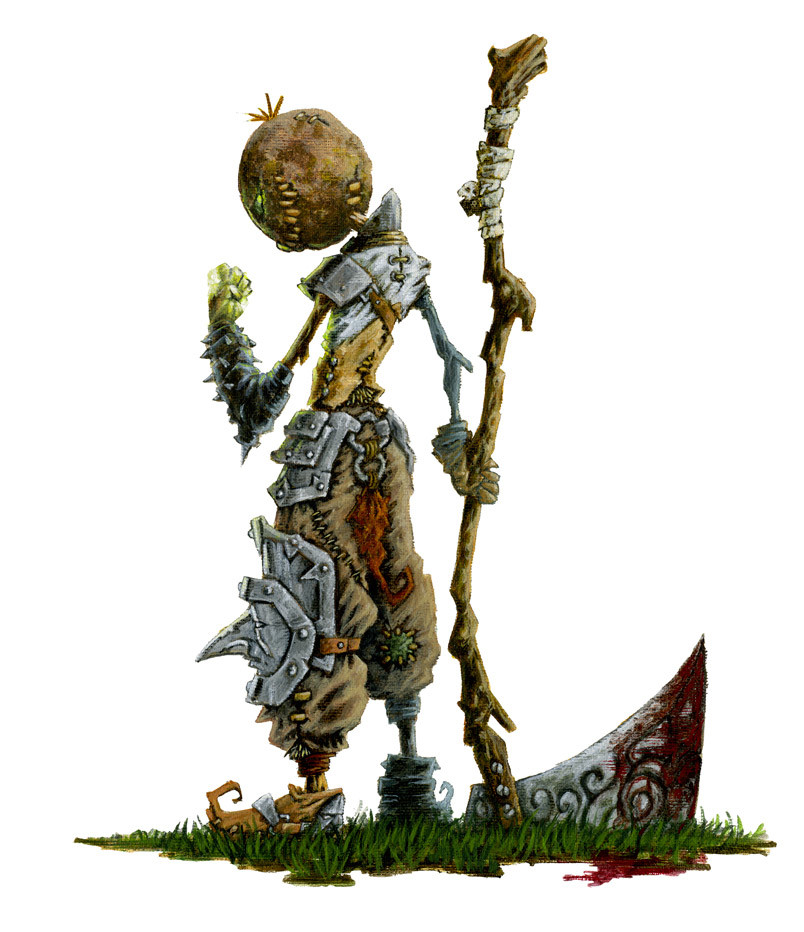This detailed illustration features a menacing character from the Kingdom Hearts franchise, inspired by The Nightmare Before Christmas. The character has a macabre form reminiscent of a scarecrow, composed primarily of sticks and possibly mud or canvas. His head, stitched together and topped with a sprig of hay, is characterized by jagged yellow teeth and a sinister smirk. His neck is a literal stick, adding to his eerie, patchwork appearance.

He is adorned in light, piecemeal armor, including metal shoulder pieces strapped over a ragged shirt and canvas. His left arm, made of sticks, is raised with a clenched fist that glows green, adorned with a sharp, spiky gauntlet. His right hand wields a massive, bloodstained scythe constructed from a rickety stick wrapped in bandages at the handle. The blade of the scythe curves dramatically with blood dried at its larger tip.

The character's tattered, patchwork pants are exceedingly baggy, and his waist is protected by loose armor connected by a chain, from which a red, tail-like sprig of hair dangles. His footwear is mismatched; the left shoe is orange with armored segments and a curled toe, while the right shoe is green, entirely cloth, and similarly curled at the toe. He stands on a patch of grass, where blood pools from his gruesome weapon.

The overall color scheme features earthy tones, with the armor rendered in steel hues, contributing to the chilling, scarecrow-like visage. The character’s back is turned toward the viewer, yet his head is turned menacingly, locking eyes with the viewer while brandishing his blood-drenched axe.